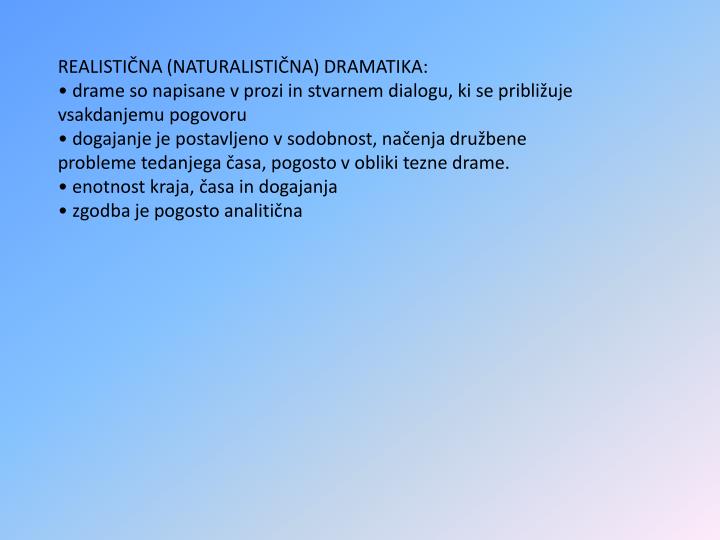This image depicts a basic presentation slide with a light blue background that gradually fades into white towards the bottom right corner. The text is left-aligned and predominantly in dark blue. The main heading at the top reads, "Realistisna (Naturalistisna) Dramatica:" in bold, capital letters. Below this heading are four bullet points, which appear to be in a foreign language and partially legible, starting with words like "drama," "do nesbist," "be person," and "in say voice." The details in the text are not entirely clear, suggesting it might be a language unfamiliar to the describers. The slide overall appears minimalist, lacking intricate graphics.